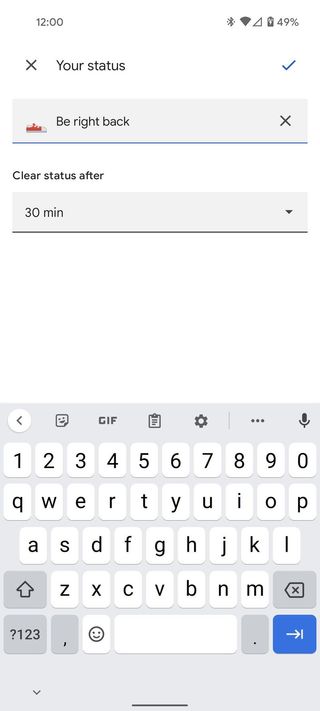The image appears to be a screenshot from a mobile phone. The status bar at the top indicates that the time is 12:00 PM, the battery level is at 49%, and both Wi-Fi and Bluetooth are enabled. Notably, there are no cellular signal bars present. Below the status bar, the screen displays a "Set Your Status" page. A text box with the pre-filled message "B right back" is visible under the header "Your Status." Below this, there is an optional setting to "Clear status after," which currently has a 30-minute duration selected via a drop-down menu. The screen's background is an all-white design, giving it a clean and minimalistic look. At the bottom portion of the image, a pop-up keyboard is shown, featuring standard letter and number keys, with options to switch to symbols. The keyboard also includes functionality for emoticons, a backspace key, and buttons to add stickers, GIFs, and access additional settings.